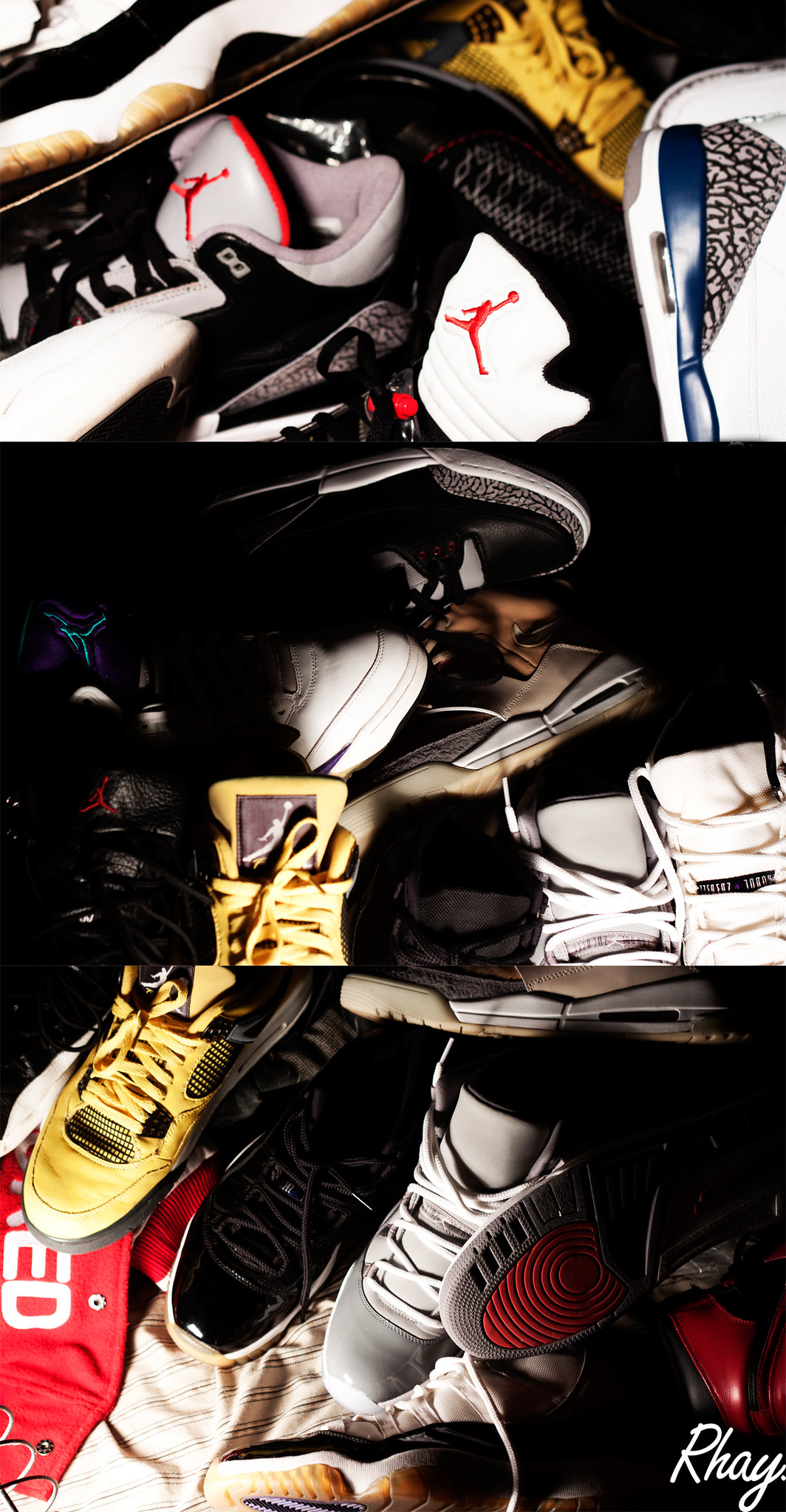This image depicts a cluttered and vertically oriented space, possibly a closet or locker, that is filled with an assortment of sneakers and athletic gear. The scene is a chaotic display with multiple colorful sneakers, primarily Air Jordans, piled together in a collage-like arrangement. The shoes are in various colors, including white, black, yellow, gray, red, and blue, often intermixed with a blanket showing hints of brown. The top section of the image is cut off, but it showcases the iconic Air Jordan logo along with the text "R-H-A-Y" written in cursive at the bottom.

On closer inspection, the space seems divided into three shelves. The top shelf appears filled with various sports equipment, including potential helmets and protective pads, characterized by a gray helmet with red and black stripes and a red logo. The second shelf is central in the image and densely packed, containing more athletic gear dominated by sneakers sprawled over the clutter. The bottom shelf distinctly displays an array of athletic shoes: a yellow shoe with black trim and laces, a black sneaker with white trim, and possibly a high-top shoe with gray and red accents. In the lower right corner, the text "R-H-A-Y" appears in italic print, adding a personal touch to this seemingly disorganized yet visually engaging depiction.